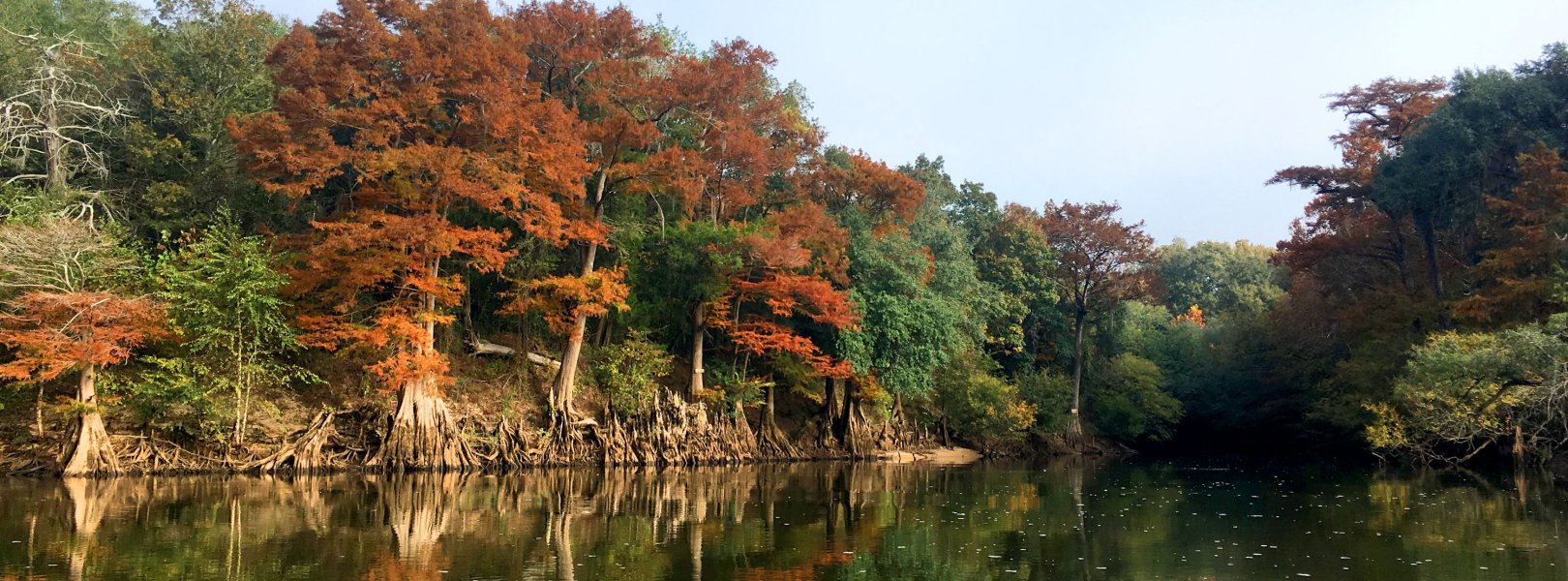A wide-angle photograph captures a serene autumn landscape, featuring a calm body of water bordered by forested banks on both sides. The scene appears to be a lake or river, with water that is a bright shade of green, reflecting the surrounding trees. The shoreline rises sharply from the edges of the water, showcasing a mix of trees, some of which are starting to turn vibrant shades of orange and red, suggestive of maple or oak trees amidst predominantly green foliage. This transition of colors signals the early days of autumn. The sky above is a clear, light blue without any clouds, adding to the tranquil atmosphere. The overall image evokes a sense of peacefulness and natural beauty, with the reflections on the still water amplifying the emotional depth and serenity of the scene.